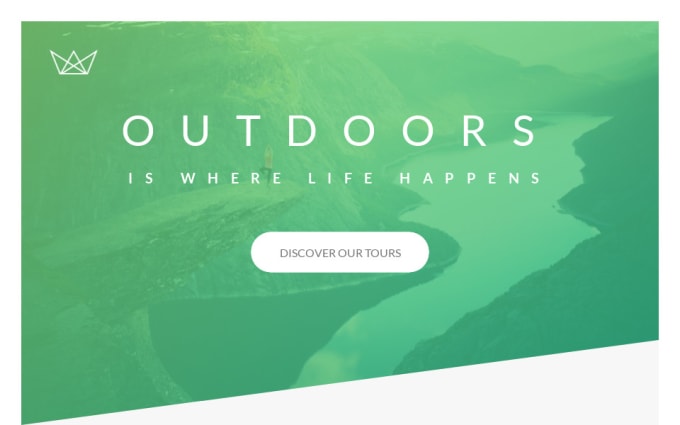This image is a partial screenshot of a tour website. The visible content primarily displays the central section of the webpage. In the top left corner of the image, there is a simplistic white drawing resembling either an origami leaf or crown. The main focus of the page features a bold statement that reads "OUTDOORS IS WHERE LIFE HAPPENS", presented in all capital letters. Directly below this text, there is a prominent white button also in capital letters, which says "DISCOVER OUR TOURS".

The background showcases an image with a green filter, making it ambiguous whether it is a photo or a drawing. This background depicts a serene scene where a person appears to be standing on a cliff, possibly in a yoga pose with one leg resting on the other. Surrounding the individual, there are mountains and a body of water, which might be a lake or a river, further enhancing the outdoor adventure theme of the website. We cannot see the top of the page, including any web links, as the screenshot focuses solely on the central content.